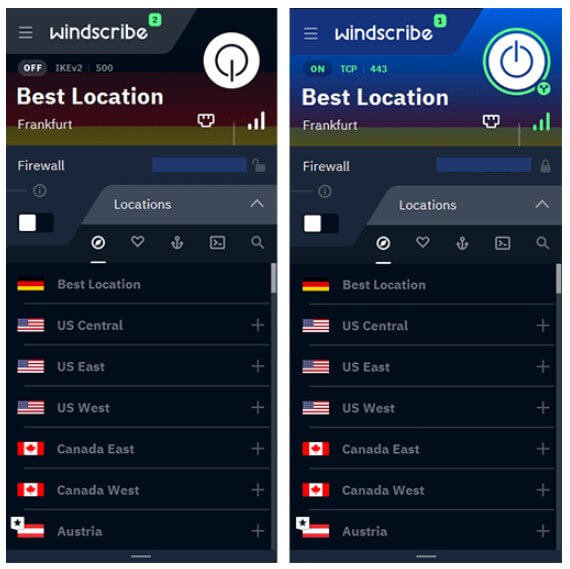The image is composed of two side-by-side screenshots, each simulating a smartphone screen displaying the WindScribe application interface. Both screenshots feature an "On" button located at the top right corner. The buttons are white and situated above a label stating "Best Location."

In the left screenshot, the "WindScribe" text is rendered in white letters within a dark blue rectangular box, set against a background that transitions from a darker to a slightly lighter blue, eventually fading into a dark purple hue.

The right screenshot presents a contrasting design, where the "WindScribe" text also appears in white but within a dark gray box. The background here starts as black at the top and gradually shifts to a deep burgundy color.

Both images indicate the selected location beneath "Best Location" as Frankfurt. Additionally, the "On" button in the right screenshot, which features the blue-purple gradient background, is highlighted with a green circle, indicating an active status. This screenshot also has additional green highlights around the top portion.

Below the primary information on both screenshots, there are lists of location options, each accompanied by the flag of its respective country. Examples include "US Central" with an American flag and "Canada East" with a Canadian flag. Both interfaces also show details labeled "Firewall" and "Locations," guiding the user through possible connection points.